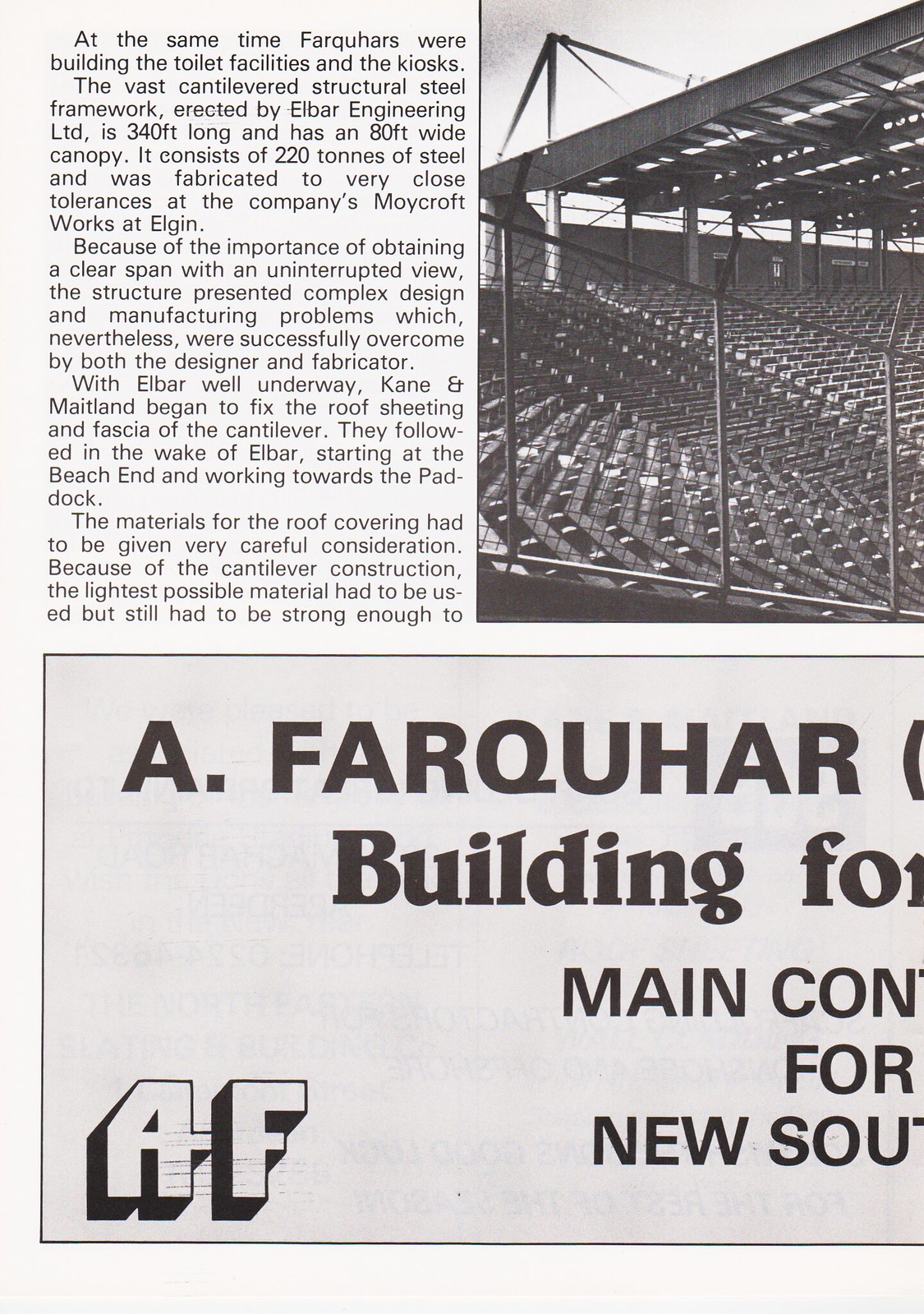The image depicts a cropped black and white page from a game day program or magazine, focusing on the construction or renovation of a soccer stadium. On the left side of the page, a column of text details the engineering efforts by Farquhar's, stating, "At the same time Farquhar's were building the toilet facilities and the kiosks, the vast cantilevered structure steel framework erected by Elbar Engineering LTD is 350 feet long and has an 80-foot wide canopy. It consists of 220 tons of steel and was fabricated to very close tolerances at the company's Moycroft works at Elgin." The upper right corner features a black and white photo showing the stadium seating and canopy under construction, suggesting the incomplete nature of the image spread. The lower half of the page, colored light blue with black print, includes an advertisement for A. Farquhar, specifying "Building 4, Main 4, New, Sow." The bottom left corner of the page displays the logo "A. F." indicating the company's branding.